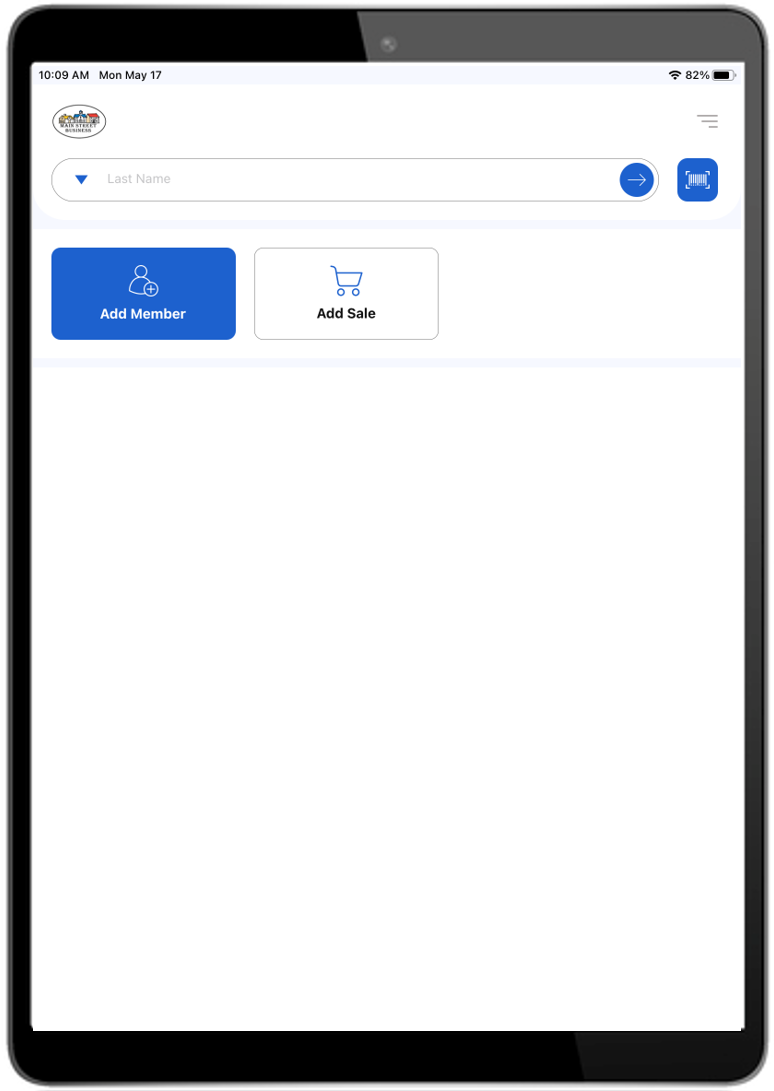The image displays the screen of a tablet, likely an iPad, showing the time as 10:09 AM on Monday, May 17th. In the top right corner, the device indicates a full Wi-Fi connection and an 87% battery life, with a battery icon visually representing the charge. 

At the top center, a small, indiscernible logo is present. Below the logo, there is a search bar with a dropdown button adjacent to it. Inside the search bar, there is a circle containing an arrow, presumably for initiating a search.

Beneath the search bar, there are two main buttons. The first button, which appears highlighted, is labeled "Add Member" and is accompanied by an icon of a faceless person. The second button, labeled "Add Sales," features a shopping cart icon. Additionally, there is a blue button, apparently for connecting to a UPC code scanner, positioned nearby.

The lower 75% of the screen is blank, save for three horizontal lines of varying lengths arranged vertically, growing longer from top to bottom. These lines likely represent a menu or additional options. The overall layout suggests a clean interface, with the content in the search bar and action buttons occupying the upper quarter of the display, while the rest of the screen remains mostly empty.